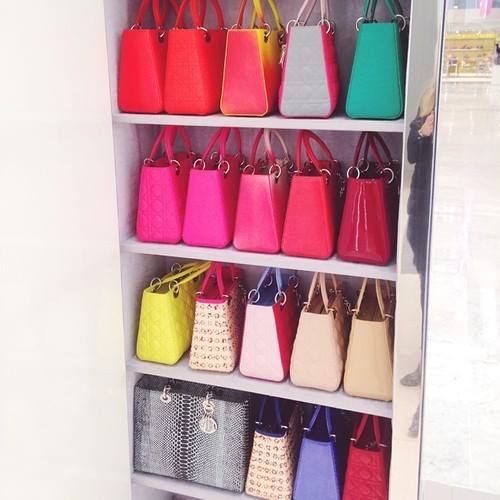The photograph captures a neatly organized display of purses on four recessed shelves, likely in a retail store or a very elegant closet. Each shelf is meticulously lined with various vibrant-colored purses, mostly designed in a Birkin bag shape. The left side of the shelves is bordered by a blank white wall, while the right side features a mirrored trim that reflects part of the photographer with blonde hair dressed in a black outfit and gray boots. Through a window beside the mirrored trim, a building with a yellow roof is visible, possibly indicating a mall setting.

From top to bottom, the top shelf features purses in shades of red, pink, a unique multicolor ombre of yellow and pink, and a striking teal one. The second shelf showcases an array of pink purses with a notable shiny red one. The third shelf includes a yellow purse, patterned purses, and several in beige tones. The bottom shelf is distinctive as one purse, exhibiting a snakeskin pattern, is positioned forward, taking up the space of two purses. This shelf also holds a blue purse, a red one, and a purple one with a patchwork texture. Overall, the harmonious blend of colors and patterns across the shelves creates a visually appealing and organized display.